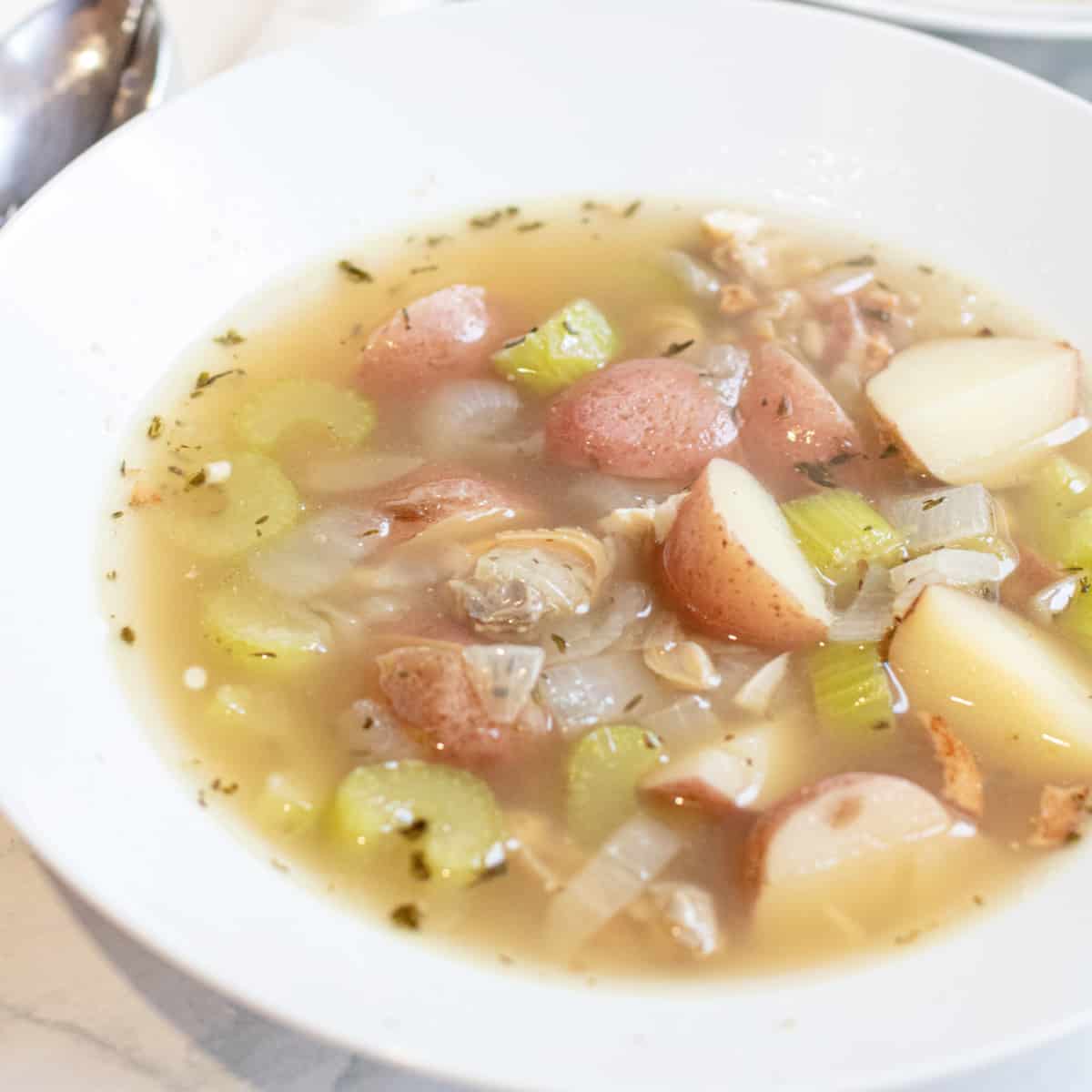This up-close image showcases a delicious bowl of creamy soup positioned in a plain, round, deep white bowl. The light yellow broth, with a hint of tannish brown, suggests it has absorbed the vibrant colors of its numerous ingredients. The soup is a hearty mix, featuring diced red potatoes, celery, onions, garlic, and possibly mushrooms and baby tomatoes. Bite-sized pieces of tender white chicken are also visible. Scattered across the surface of the soup are tiny specks of herbs and spices, such as basil, fennel, oregano, or thyme, adding a flavorful touch. Behind the bowl, you can see the tip of a small silver spoon resting on what appears to be a white tabletop or tablecloth. The entire composition is framed within a rectangular image.